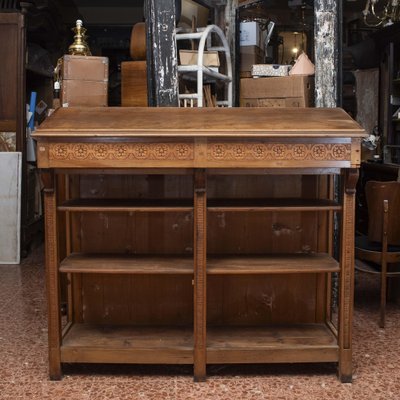The image features an intricately designed antique wooden console table, prominently situated in what appears to be a cluttered, old storage unit or possibly an antique store filled with various vintage items. The table itself is characterized by its shiny, polished surface and detailed carvings, with circular floral designs adorning its edges. Below the smooth wooden top, the console table is structured with three open shelves that run its length, ideal for displaying items such as cookbooks or sculptures. The floor beneath is brown marble, adding to the antique ambiance. Surrounding the central piece are numerous other old furniture items, including a trunk, a white table, and a chair, all contributing to the overall busy and nostalgic atmosphere.